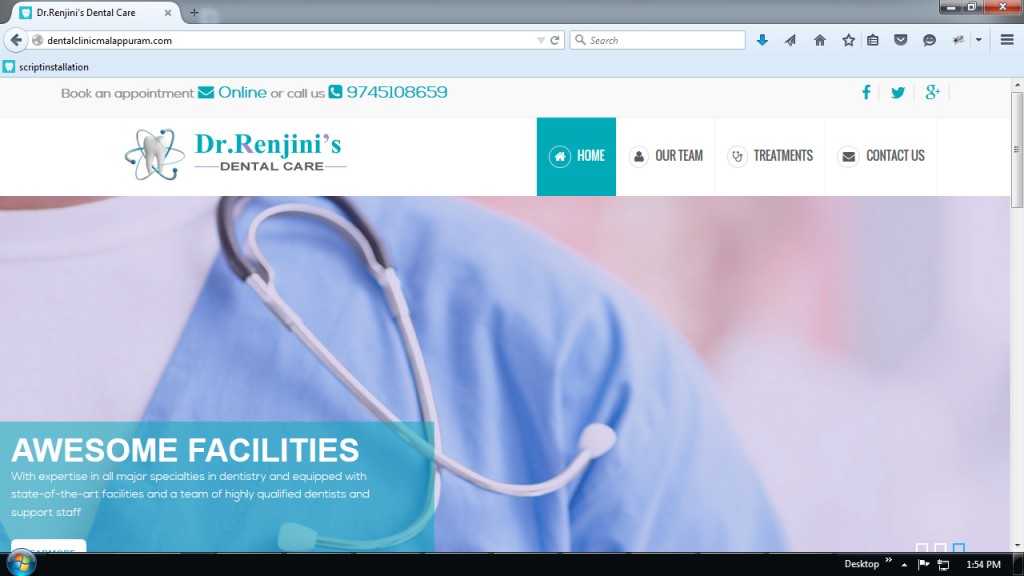The image depicts the homepage of Dr. Rangini's Dental Care website. Dominating the top part of the page is a white banner featuring teal and black lettering. The banner encourages visitors to "book an appointment online or call us." 

Embedded within the banner on the left-hand side is a close-up photograph of a doctor, showing their shoulder and chest area adorned with a stethoscope draped around their neck. The ear plugs of the stethoscope are clearly visible in the image. 

In the lower left-hand corner of the banner, a text box highlights the clinic's attributes, stating, "Awesome facilities with expertise in all major specialties in dentistry and equipped with state-of-the-art facilities and a team of highly qualified dentists and support staff."

At the top of the website, navigational links including "Home," "Our Team," "Treatments," and "Contact Us" are displayed, along with icons for Facebook, Twitter, and Google Plus, suggesting the clinic's presence on social media platforms.